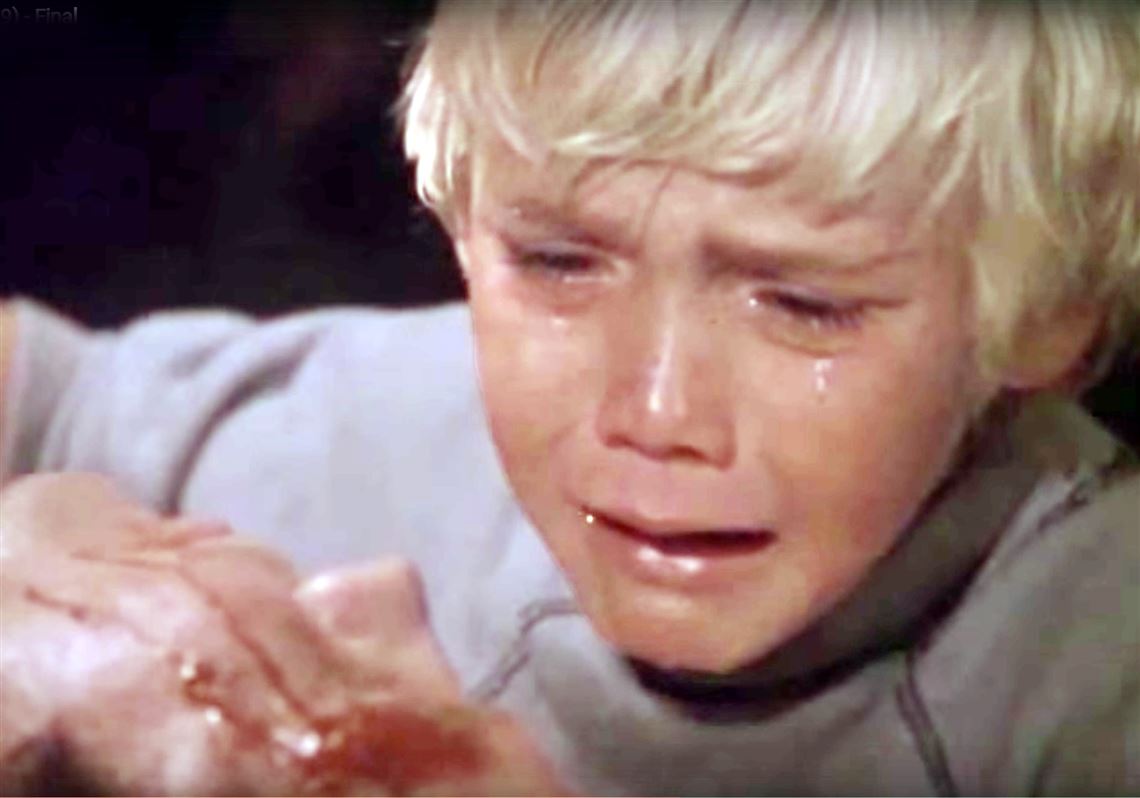The image, a grainy and blurry screenshot likely from an old movie or television program, dating possibly from the 1960s, captures a highly emotional scene featuring a young Caucasian boy, around 11 or 12 years old, with blonde hair. The rectangular frame, measuring about six inches wide by four inches high, focuses primarily on the boy's head and shoulders, with the top of his head slightly off-screen to the right. He is wearing a light gray long-sleeved shirt and is visibly distraught, with tears streaming down his cheeks and his mouth open in an expression of sorrow. The boy is looking downward towards the bottom left of the image, where he appears to be holding up his hand or part of his arm, which shows a small red blister that could signify blood. The background on the upper left corner is darkened to black with bits of brown, adding to the somber tone. Additionally, there is a partial side view of a person's face lying down in the lower left corner, also appearing to have blood on it, likely contributing to the boy's distress. This intense moment captures a poignant and dramatic narrative from the visual media of its time.